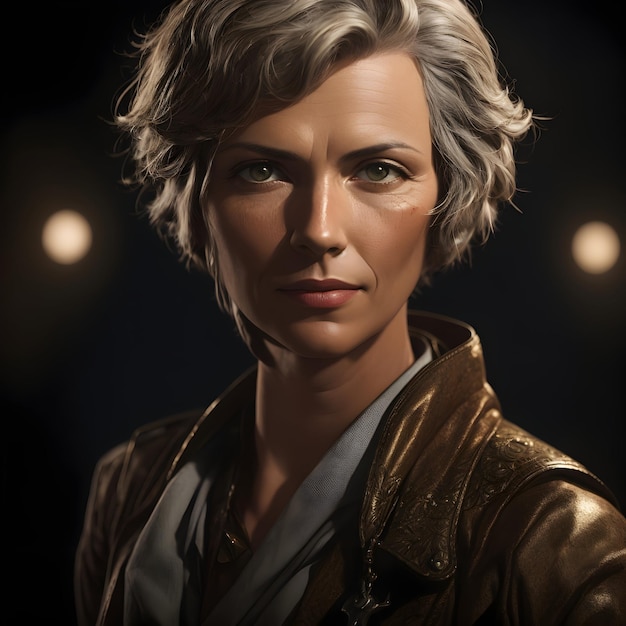This image features a computer-generated portrait of a young woman with platinum-colored hair and striking green eyes. Her expression is stern, evoking a sense of determination and resilience. She is dressed in a brown leather jacket with a high collar, underneath which she wears a gray scarf and a dark shirt. The background is entirely black, contrasted only by two round orbs of light positioned symmetrically on either side of her head. This minimalistic setting, combined with the lighting from the upper right that casts a shadow on the left side of her face, enhances her enigmatic and commanding presence. The image suggests a character who might be a superhero or a video game protagonist, one who seems poised for action in a dark, mysterious environment.